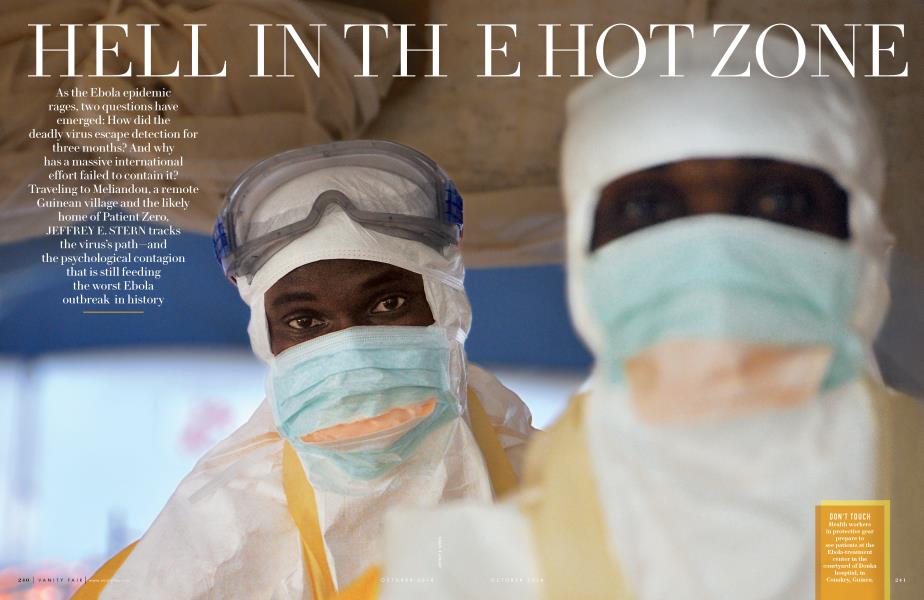The image resembles the cover of a high-profile magazine, meticulously designed to capture attention. At the forefront, two individuals with dark complexions are prominently featured, both adorned in surgical masks and caps, indicating a medical or emergency setting. Their ears are covered with white protective gear, and the person on the left additionally wears clear plastic safety glasses, enhancing the impression of a high-stakes environment.

The bold white headline, "Hell in the Hut Zone," dominates the upper part of the cover. Notably, the word "Hell" is separated from "The" in a visually striking manner, with "In" placed between them, followed by "Hut Zone." The layout creates an arresting visual effect, drawing the reader's eye and accentuating the headline's urgency.

In the bottom right-hand corner, a small column of text is set against an orange background, bordered on the top and right side with yellow. While the text itself is illegible, its distinct placement and coloring likely indicate additional important information or a teaser for the magazine's content. This detailed and thoughtfully arranged cover successfully piques interest while conveying a sense of urgency and significance.